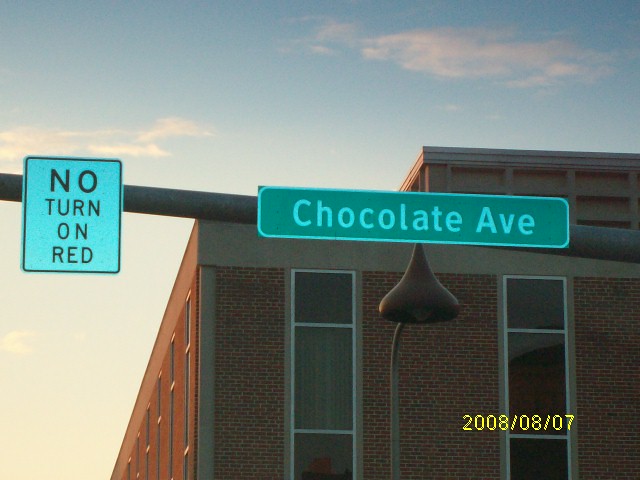This photograph captures a green rectangular street sign with white trim and lettering, displaying "Chocolate Avenue." The sign is affixed to a high, horizontal metal pole positioned above the street. Directly behind it, a streetlight mounted on a silver pole features a unique Hershey's chocolate drop-shaped lamp. To the left of the Chocolate Avenue sign, another rectangular sign with a black border reads "No Turn on Red" in black letters. In the background, a tall multi-story red brick building with long vertical windows stands prominently. The sky is a clear blue with a few faint white clouds. A timestamp at the bottom indicates the photo was taken on August 7, 2008.